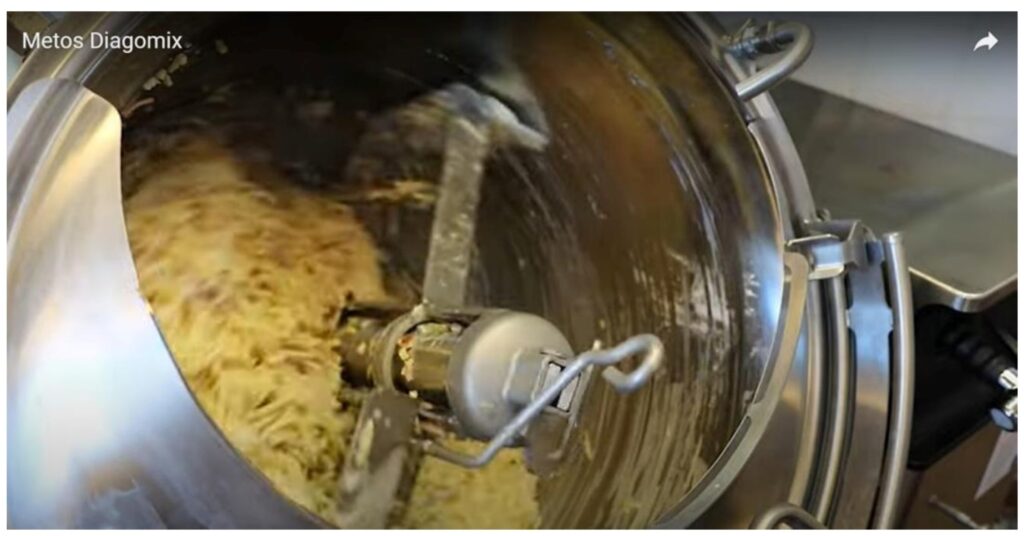The image depicts a Meadows Dye Agamix, an immense industrial-strength mixer designed for heavy-duty tasks. Constructed entirely from stainless steel, this formidable machine rests directly on the floor, underscoring its substantial size and weight. The mixer is captured at an angle, revealing motorized beaters that reach deep into the mixing bowl. These beaters scrape along the sides as they rotate, efficiently kneading what appears to be dense, stretchy dough—likely bread dough, given its texture. The mixer is paired with an adjacent table on the right and features a hook attachment, presumably used to extract the substantial dough from the bowl, which would be a challenging task without such an aid. The interior of the bowl is slightly blurry, suggesting the vigorous motion of the beaters working the dough. The overall impression is one of robust industrial capability, suited for large-scale baking operations rather than typical home use.